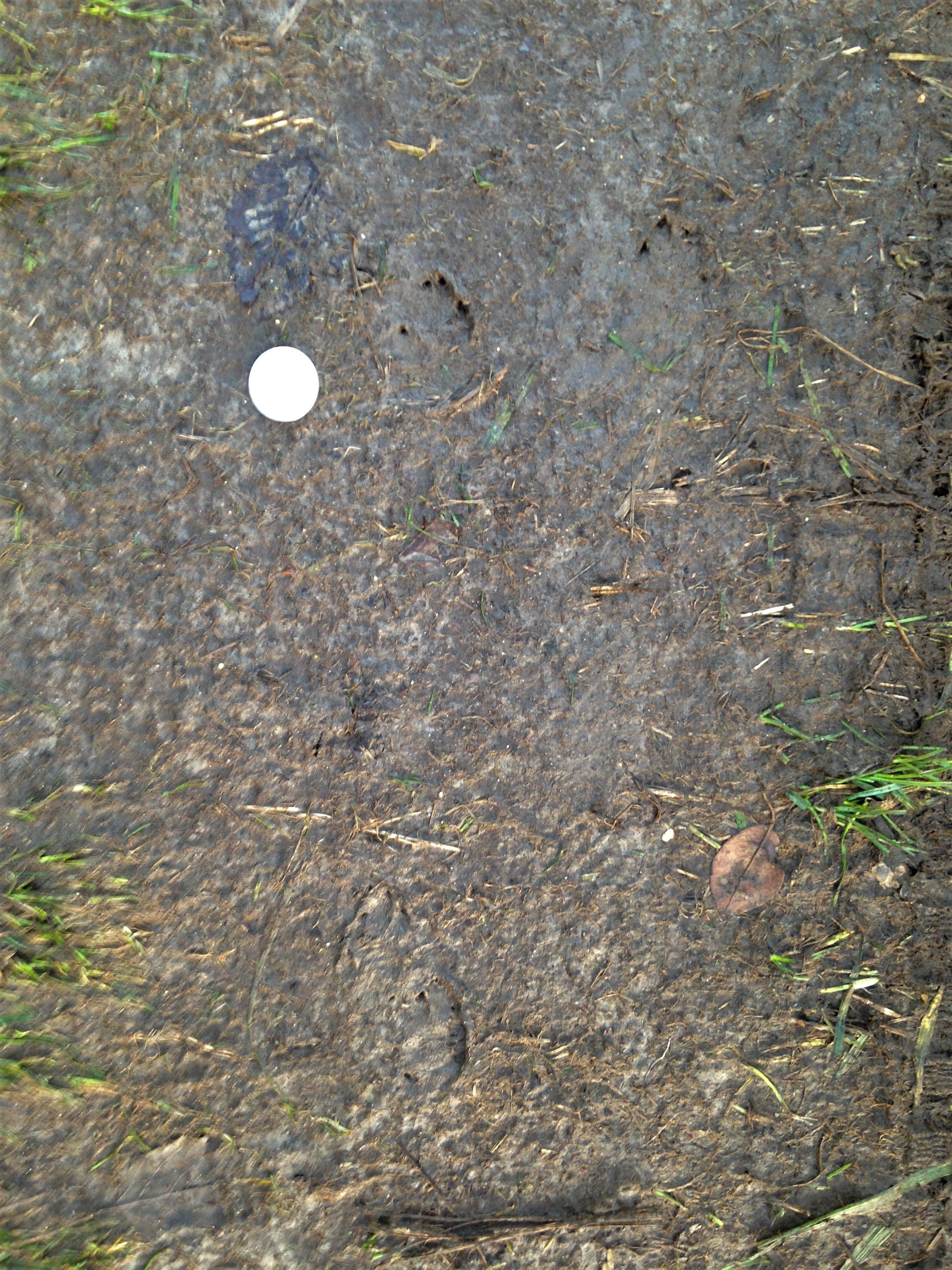The image depicts an aerial view of a muddy, almost desolate patch of ground, possibly resulting from a recent rain. The surface is largely covered in solid, mushy dirt with a few scattered footprints indicating someone might have walked through and got the bottom of their shoes or boots muddy. Strands of grass and weeds are visible, primarily on the periphery—specifically in the upper left, bottom right, and bottom left areas. Notably, there's a white, circular object in the upper left quadrant that could be a piece of discarded garbage, perhaps the lid of a jar. The landscape is interspersed with various organic debris, including a dark brown or black leaf and several sticks and twigs, contributing to the overall impression of a washed-out, neglected area.